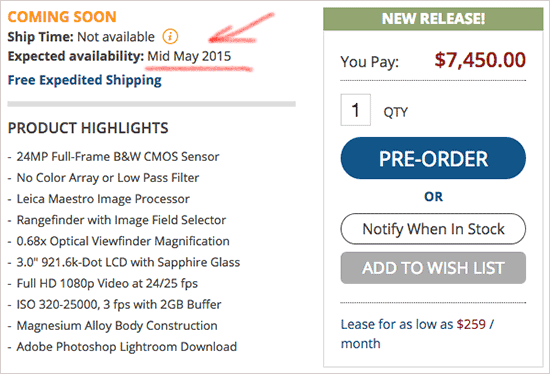The image displays a cropped section of a website, showcasing a product listing with a predominantly white background. At the top left, an orange header reads "Coming Soon," followed by a notification in regular text stating, "Ship time not available, expected availability mid-May 2015." This notice is underlined in red with an arrow pointing to it, added post-image creation for emphasis.

Beneath this section, the text "Free expedited shipping" appears in blue font. Below it, the product highlights are listed, detailing the features of a high-end camera. These include:

- A 24 MP full-frame B&W CMOS sensor without a color array or low-pass filter,
- Leica Maestro image processor,
- Rangefinder with an image field selector,
- 0.68x optical viewfinder magnification,
- 3-inch 921.6K dot LCD screen protected by sapphire glass,
- Full HD 1080p video recording at 24-25 frames per second,
- ISO 320 to 25,003 FPS with a 2GB buffer,
- Durable magnesium alloy body construction,
- Adobe Photoshop Lightroom download included.

The product is identified as a new release, priced at $7,450, with an option to pre-order or to be notified when it is back in stock. Alternatively, buyers can add the item to their wish list using the button below the listing. Additionally, there's a leasing option available for as low as $259 per month. This section clearly indicates options for pre-ordering or purchasing the product.